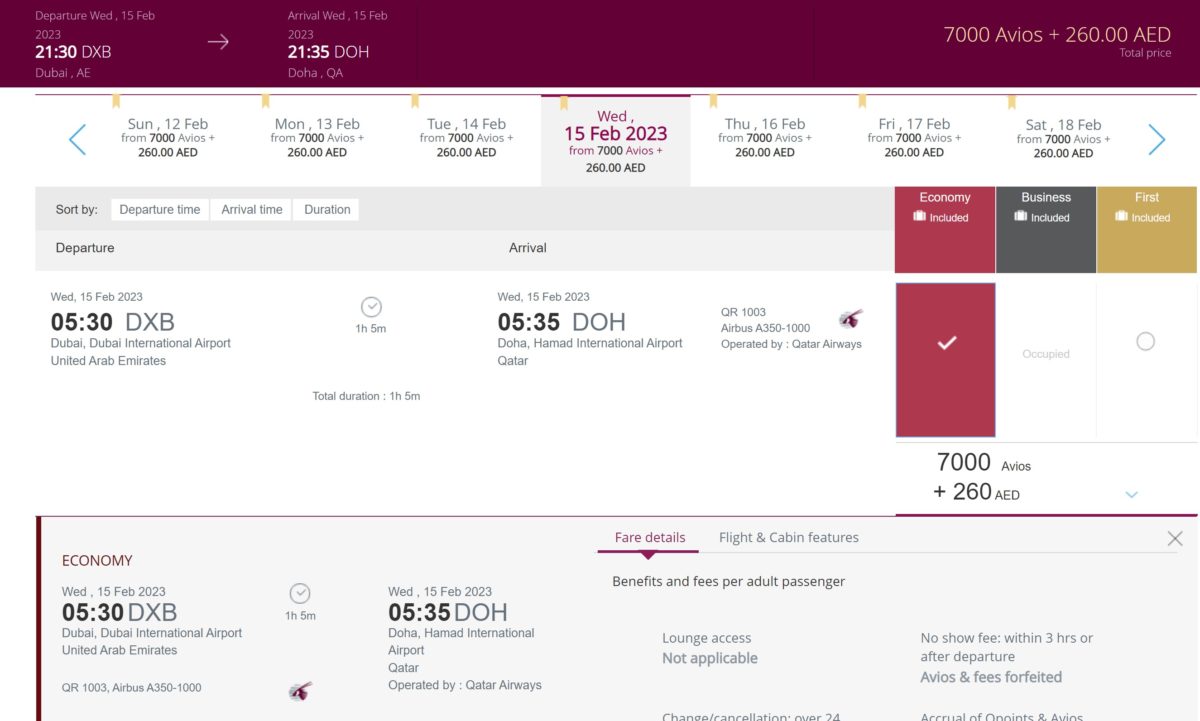This is a detailed screenshot of a flight booking page, highlighting a specific airfare option. At the top, a bright red box with pink and white lettering displays essential flight information. The departure is scheduled for Wednesday, February 15, 2023, at 21:30 from Dubai (DXB). The arrival time is listed as the same day, February 15, 2023, at 21:35 in Doha, Qatar (DOH), which indicates an hour time difference and suggests an actual flight duration of approximately one hour and five minutes.

The cost for this flight is detailed as 7,000 Avios points plus an additional AED 260.00. Beneath this primary option, the website displays alternative flight dates ranging from February 12 to February 18, with the same pricing for each day.

Further details include a secondary departure option at 05:30 from Dubai International Airport (DXB), arriving at 05:35 in Doha, Hamad International Airport (DOH), again implying an hour and five-minute flight considering the time difference. The flight is operated by Qatar Airways using an Airbus aircraft.

At the bottom, the screenshot provides information on the benefits and fees per passenger, including lounge access, and outlines the no-show fee policy: Avios points and fees will be forfeited if the no-show occurs within three hours before or after the scheduled departure.